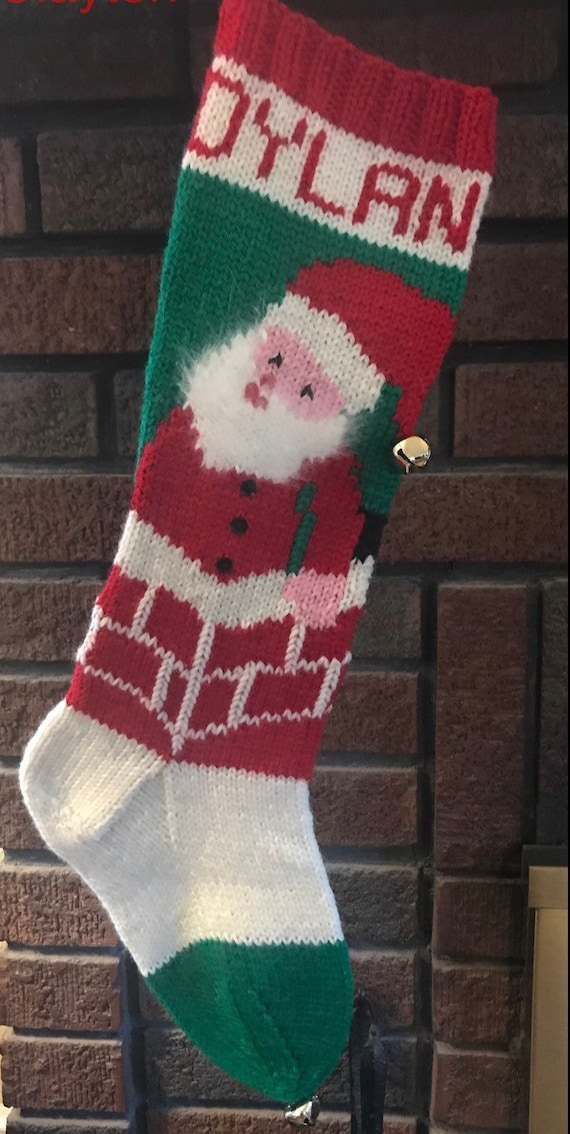Hanging on a red brick fireplace with a golden metal front, there is a detailed Christmas stocking. The stocking has a red band at the top, followed by a white band with the name "Dylan" written in red letters. Below this is a green band featuring an image of Santa Claus emerging from a red chimney. Santa is depicted in his traditional red outfit, complete with a red hat that has a white puffball and a tiny gold jingle bell. Santa’s fluffy white beard and red lips complement his white skin. The toe section of the stocking is green and white, and another jingle bell is attached at the tip. The background behind Santa is green, and the overall image includes a color block design with sections of white and green. Fireplace equipment is visible near the hearth, completing the cozy, festive scene. The image captures a classic indoor holiday moment with intricate details on the stocking and a warm, welcoming fireplace.